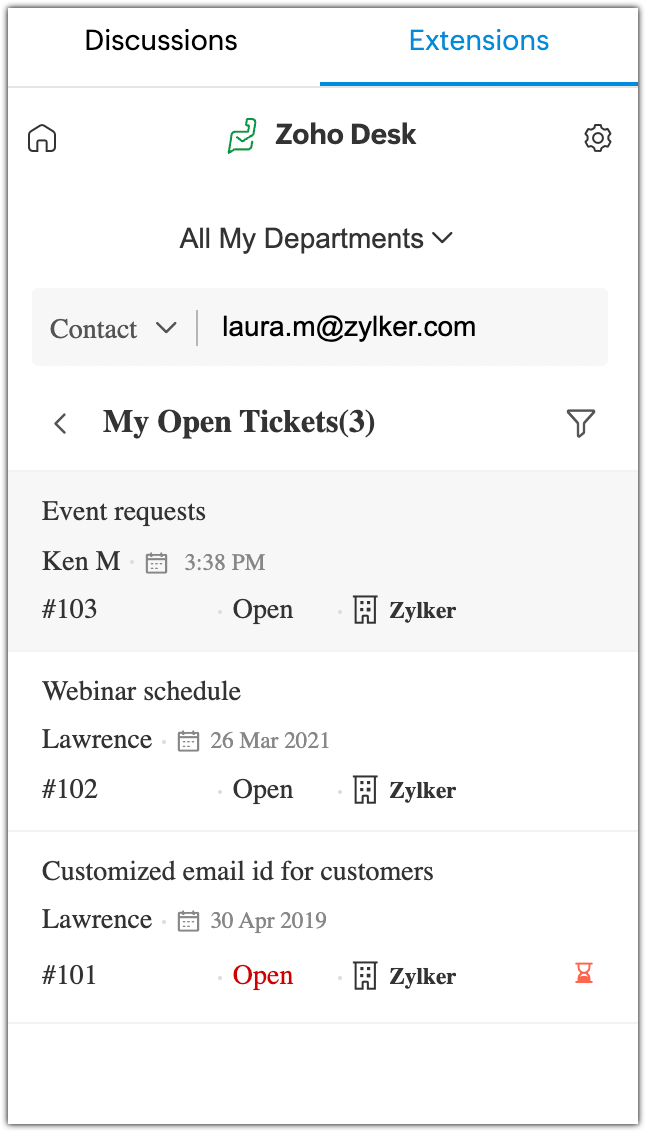The image depicts a Zoho Desk dashboard interface. At the top, there are two selectable tabs: "Discussions" on the left and "Extensions" on the right. The "Extensions" tab stands out as it's blue and underlined, indicating it is currently active.

Below the tabs, "Zoho Desk" is prominently displayed in bold black text. To the right of this heading is a settings icon, and to its left is a home icon. Beneath this, the text "All my departments" appears with an option to expand, followed by a contact section displaying an email address, laura.m@zilker.com, alongside an expandable option.

Further down, the section titled "My Open Tickets" is highlighted in bold black, with a total count of three indicated in brackets. The first ticket is for "Event Requests" assigned to Ken M., marked as number 103, and timestamped at 3:38 PM. It is tagged as "open" and labeled "Zilker."

The second ticket concerns a "Webinar Schedule," assigned to Lawrence, dated March 26th, 2021, and marked as number 102. It is also open and labeled "Zilker."

The third ticket addresses "Customized Email ID for Customers," assigned to Lawrence, dated April 30th, 2019, and identified as number 101. Unlike the others, "open" is written in red, indicating urgency or a different status. This ticket also has an hourglass icon in red at the bottom right corner, symbolizing a time-related priority or overdue status.